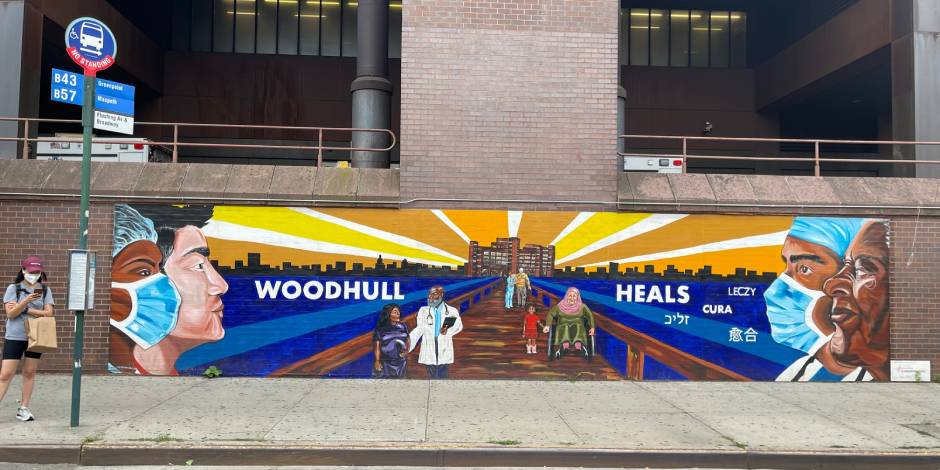This photograph, taken outdoors, captures a wide scene with vivid detail. On the far left, a woman wearing a gray short-sleeved shirt, black shorts, white shoes, a burgundy hat, and a white face mask stands on a concrete sidewalk, holding a brown paper bag. She is looking down at her phone beside a street sign indicating "No Standing" and bus routes B-43 and B-57.

To the right of her, past a bus stop sign, there is an elaborate mural painted on a brown brick wall. The mural prominently displays the words "Wood Hole Heels" in white lettering. It features a vibrant scene of medical providers and health care workers. Close-up portraits of doctors in surgical caps and masks flank the mural on both sides. Within the mural, various figures including doctors, an Asian man in a surgical mask, a black doctor in a white coat, a woman in a wheelchair wearing a green dress, and a little girl in a red outfit are depicted walking along a wooden boardwalk. This boardwalk leads towards a large hospital in the distance, from which beams of white light interspersed with yellow and orange hues radiate. 

Above the mural, the large building in the background, likely the actual hospital, features many rows of windows. On an upper level, an ambulance is parked, suggesting a hospital parking lot. The photograph ingeniously captures the essence of community and healthcare amidst a cityscape backdrop.